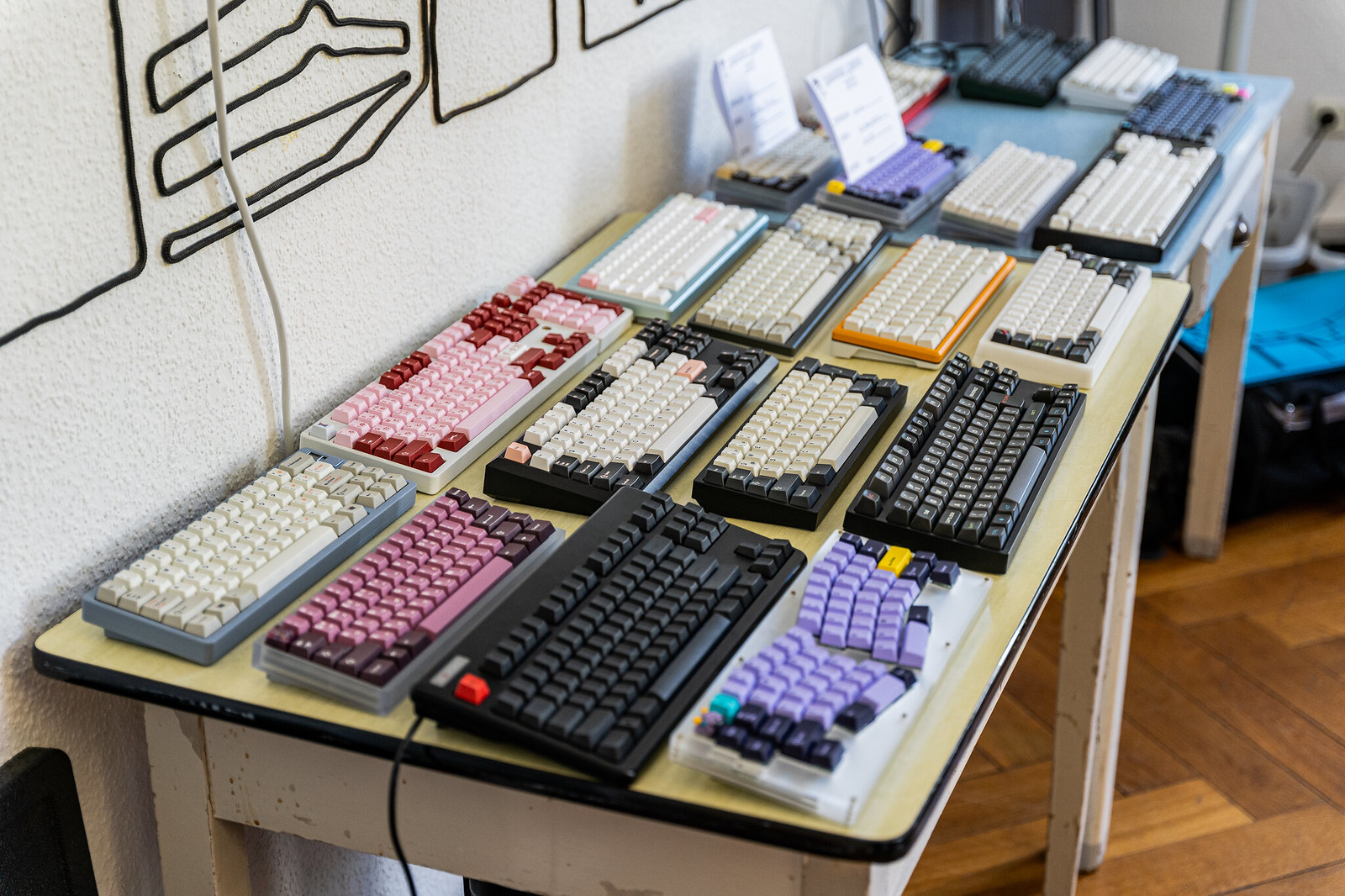The photograph showcases an eclectic collection of around 20 computer keyboards arranged on two adjacent tables against a white wall featuring black wire grid designs. The main off-white, rectangular table with six legs displays twelve keyboards, while the smaller, square table with a light blue top and a drawer underneath holds eight keyboards. The keyboards vary widely in both color and design, showcasing hues of black, white, pink, purple, red, blue, light gray, dark blue, and even yellow. Notably, one keyboard in the front with purple and black keys appears broken, with a distinctive dip in the middle, suggesting a unique ergonomic design. These keyboards are compact, mostly lacking numeric keypads and function keys, and they resemble old-style mechanical click keyboards. The tables are situated on a brown parquet wooden floor, and the overall variety and arrangement of keyboards create an intriguing and colorful display.